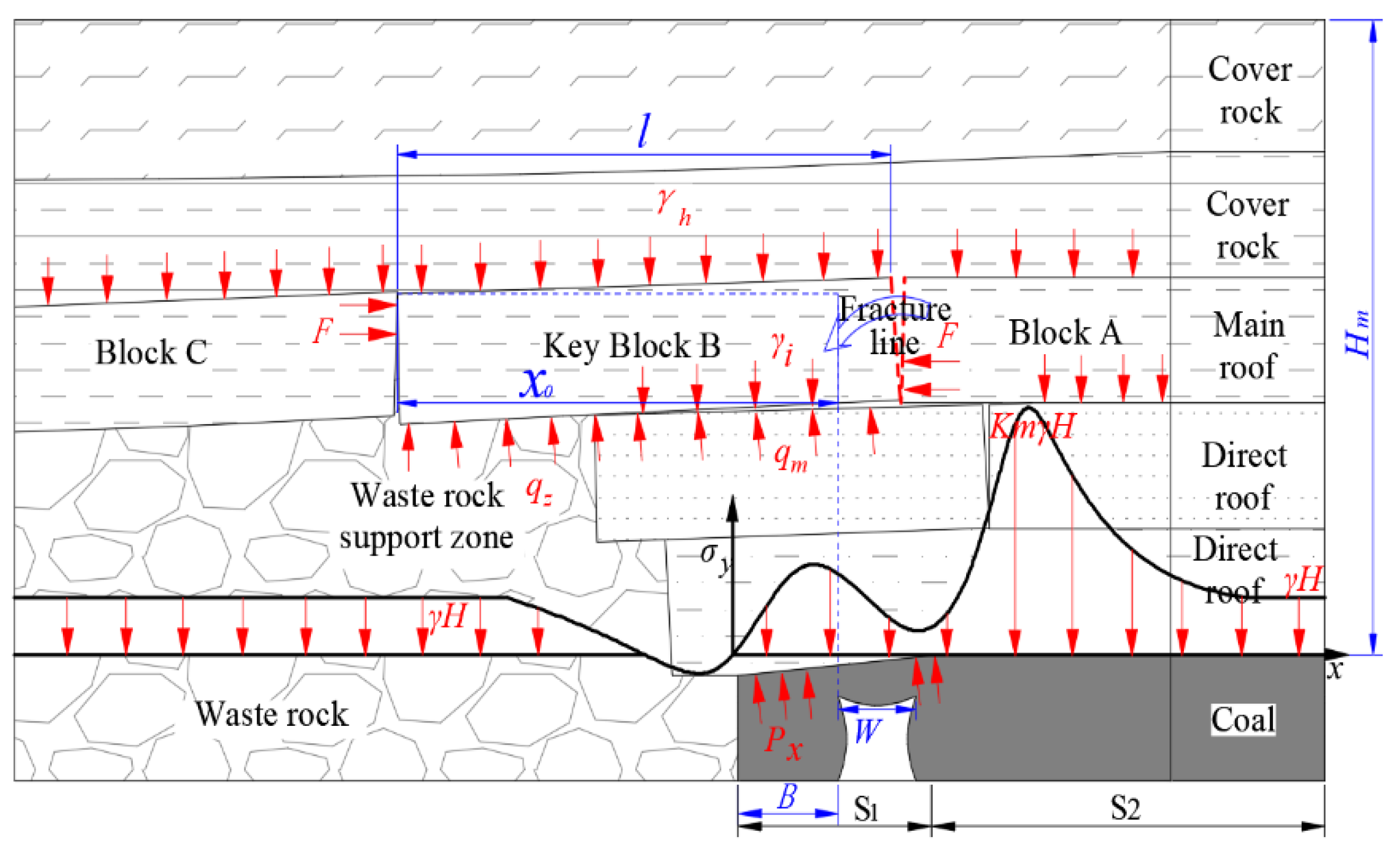This infographic is a detailed, line-drawn cross-sectional diagram related to coal mining, illustrating various geological layers from top to bottom. The image is outlined in black with black text and features red and blue arrows and insets.

At the top, there are two layers labeled "cover rock," both depicted with a slanting slightly downward line towards the left. Below these layers lies the "main roof," which is divided into three distinct blocks: Block A, Block B, and Block C. A fracture line separates Block A and Block B. Surrounding the main roof are arrows with labels: red arrows pointing downward labeled "YH," and arrows labeled "FF" pointing in from both sides. From the bottom of the main roof, there are upward-pointing arrows labeled "Q" and "QM."

Beneath the main roof is the "direct roof," depicted in two levels, with a dotted panel and a rocky textured panel labeled "waste rock support zone." Further down is a layer marked "waste rock," characterized by various-sized rocky textures and red arrows labeled "YH" pointing downward.

In the lower sections, the rightmost area shows a "coal" layer shaded in gray, featuring a magnified blue inset in the lower right corner. This coal segment includes a bag-like design labeled "W" with blue arrows. Additionally, the coal section's bottom part is divided into sections labeled "S2," spanning a short distance, and "S1," before another section labeled "B" with a blue arrow.

The detailed layout and these distinctive markers emphasize water flow and structural support within this geological slice, providing a comprehensive view of the layers and their characteristics.